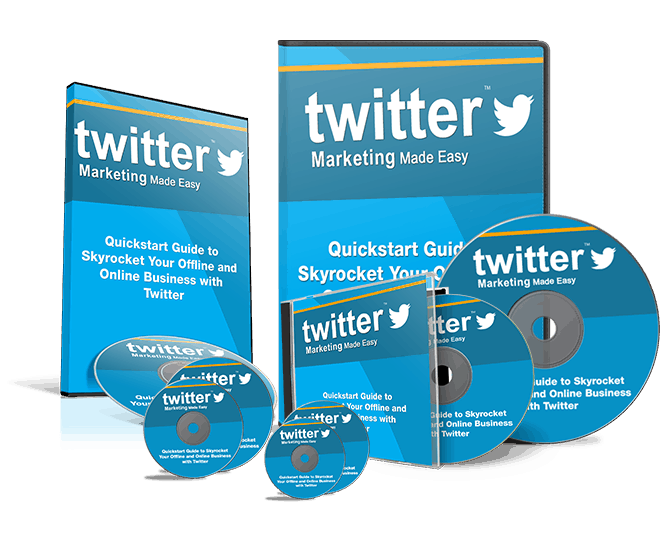The image showcases a collection of marketing materials for Twitter, displayed against a white background. There are a total of 10 items, which include 3 DVD packs and 7 individual DVDs/CDs. Each disc is circular and prominently features the Twitter logo, a bird symbol, and a trademark icon positioned to the right of the word "Twitter." The text on each item reads, "Twitter, Marketing Made Easy: Quick Start Guide to Skyrocket Your Offline and Online Business with Twitter." The materials are designed in a color palette comprising blue, black, yellow, and white.